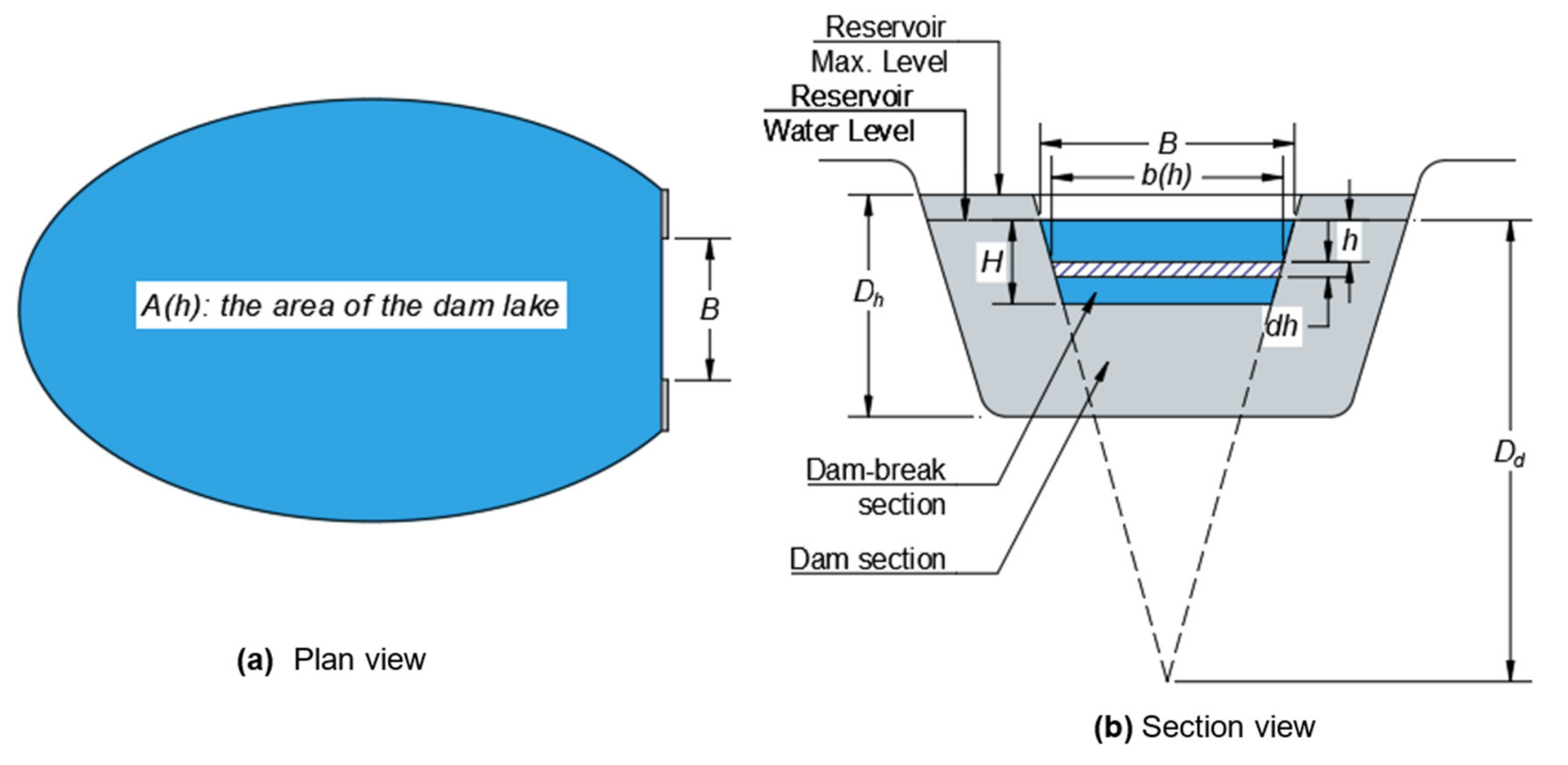This is a detailed diagram illustrating the structural and sectional views of a dam and its associated reservoir. 

On the left side, labeled as "Plan View (A)," a blue partially oval shape represents the area of the dam lake. This oval is truncated on the right side and denoted by the text "AH, the area of the dam lake," written in dark blue or black. At the top and bottom of this shape, two gray rectangles are connected by vertical arrows, with a central black letter "B" indicating the width between the rectangles.

On the right side, designated as "Section View (B)," the diagram details a cross-sectional view of the dam. The gray, bowl-like structure contains various arrows and measurements. A blue section signifies the water level within the reservoir. Key labels include "Reservoir Max Level" and "Reservoir Water Level." Measurements are marked with various letters such as B, b, H, h, and dH, indicating widths and heights.

Additionally, the diagram includes terms like "Dam Break Section" and "Dam Section," each pointing to specific parts of the gray structure. Vertical and horizontal lines with arrows illustrate various dimensions, such as D and d, which are used to measure heights and other critical aspects of the dam’s structure.

Overall, the diagram employs blue, gray, and white colors to differentiate between the water, structural elements, and background, providing a comprehensive guide to understanding the dimensions and functional components of the dam and reservoir system.